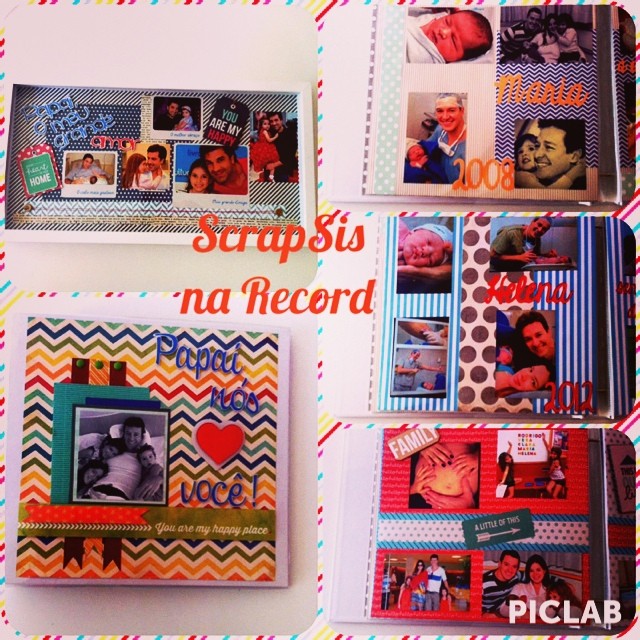The image displays a collage of scrapbook pages, adorned with various family photos and vibrant decorations on an off-white background. The border of these pages is sprinkled with colorful accents in pink, yellow, and blue. Central to the image is an orange-tinted text watermark that reads "Scrapsis Na Record," which is slightly obscured by the surrounding elements.

On the left side, there are photos featuring a man and his daughter, with him holding her in a sequence of five pictures. Stickers embellish these images. To the right, there are additional photos with captions such as "Maria 2008" in orange writing and "Helena" in red writing, alongside several pictures of babies and parents. A bottom photo with the caption "family" shows someone pregnant and family members surrounding them. Additionally, the lower left corner has the words "PAP I A," a heart symbol, and "VO CE," depicting a family laying together. Lastly, the bottom right corner of the image is marked with “PicLab” in white, indicating the editing tool used.

The image contains a mix of Polaroid-style photos and actual pictures, each capturing precious family moments, suggesting these are sentimental scrapbook pages likely created to cherish memories of familial bonds and milestones.